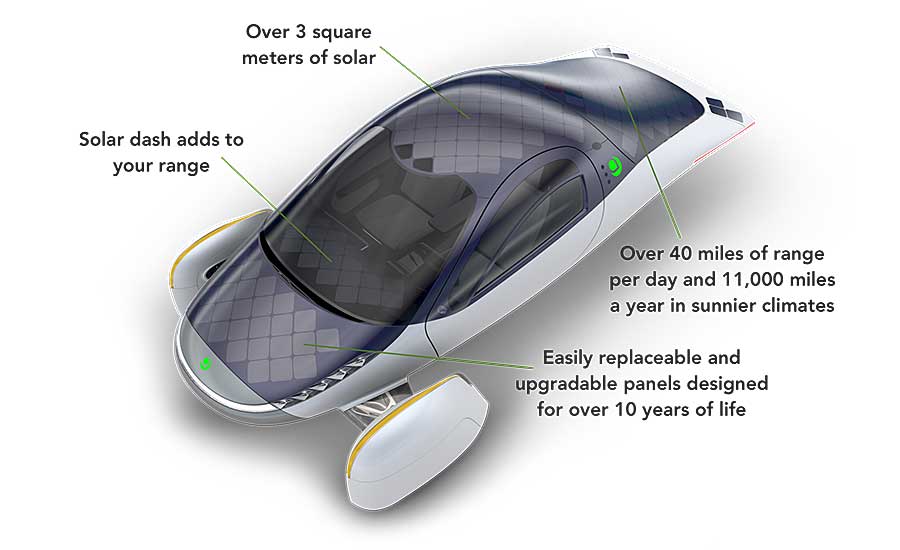This 3D digital rendering showcases a sleek, futuristic prototype vehicle prominently featuring advanced solar technology. The car's design is smooth and curved, incorporating translucent glass elements that reveal white seats inside. The chassis appears mainly white with accents of blue, encapsulating a high-tech aesthetic. The front wheels are encapsulated in a white enclosure accented with yellow strips, suggesting a unique wheel configuration that might include just one rear wheel, contributing to its avant-garde look. 

The vehicle is heavily integrated with solar panels, as indicated by various annotations pointing to different sections. On the roof, a label reads "over three square meters of solar," highlighting the large solar panel array designed to harness maximum sunlight. These panels extend to the vehicle's dash, with a note that reads "solar dash adds to your range," suggesting additional solar panels embedded in the windshield area. On the body below the roof, a marker states "over 40 miles of range per day and 11,000 miles a year in sunnier climates," indicating the significant travel range afforded by its solar capabilities. Additionally, the hood features a note, "easily replaceable and upgradable panels designed for over 10 years of life," emphasizing the durability and modularity of the solar components. This vehicle design prioritizes sustainability, extended range, and long-term use, encapsulating the future of eco-friendly transportation.